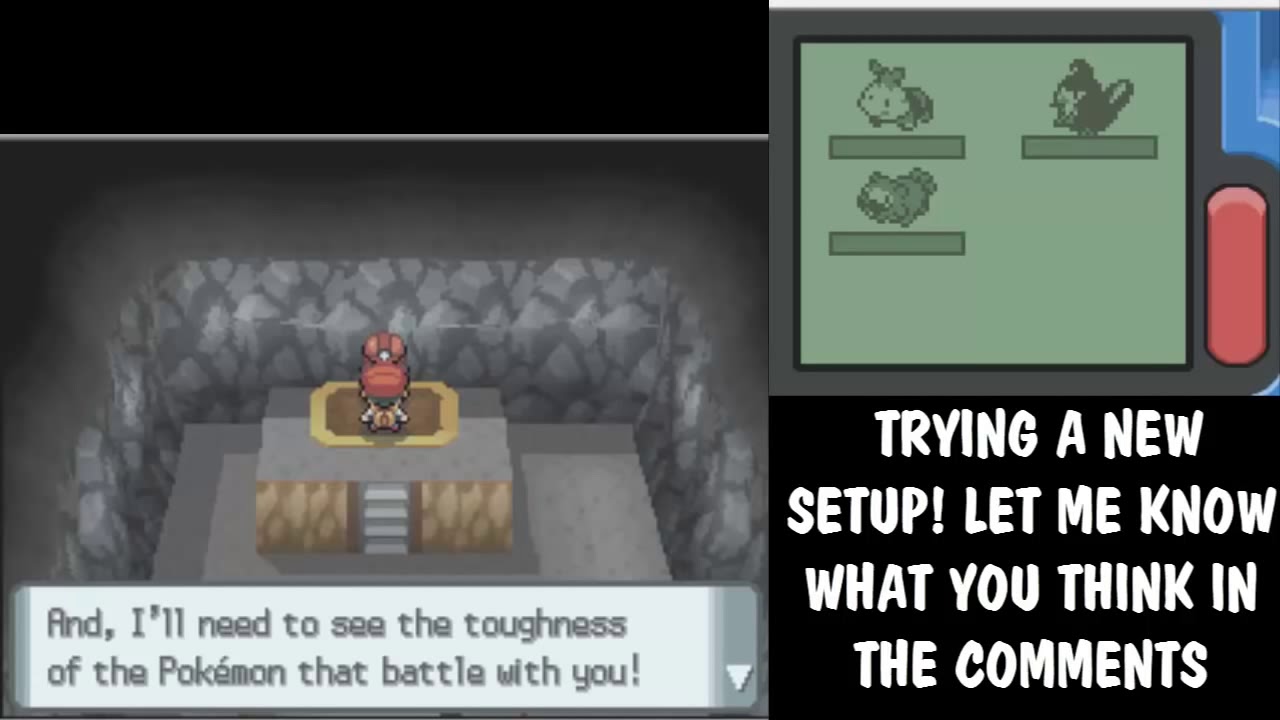The image appears to be a screen capture from a retro-style video game, reminiscent of the Super Nintendo era with detailed 16-bit graphics. The screen is divided into distinct sections, with approximately 60% on the left showing a small character with red hair standing on a raised platform, in what seems to be a cave environment surrounded by gray stone walls. There is a stairway leading up to where the character is standing. A black bar spans across the top 20% of this left section, containing a text box that reads, "I'll need to see the toughness of the Pokémon that battle with you."

The right 40% of the screen features a smaller section with an LED display showcasing different Pokémon, each with health bars visible. Below this display, there is a black box with white text that reads, "Trying a new setup. Let me know what you think in the comments." A red button is also present to the right of the LED display. Overall, the image captures a nostalgic, pixelated aesthetic typical of classic Pokémon games, complete with on-screen text and various interface elements indicating a setup or configuration process.